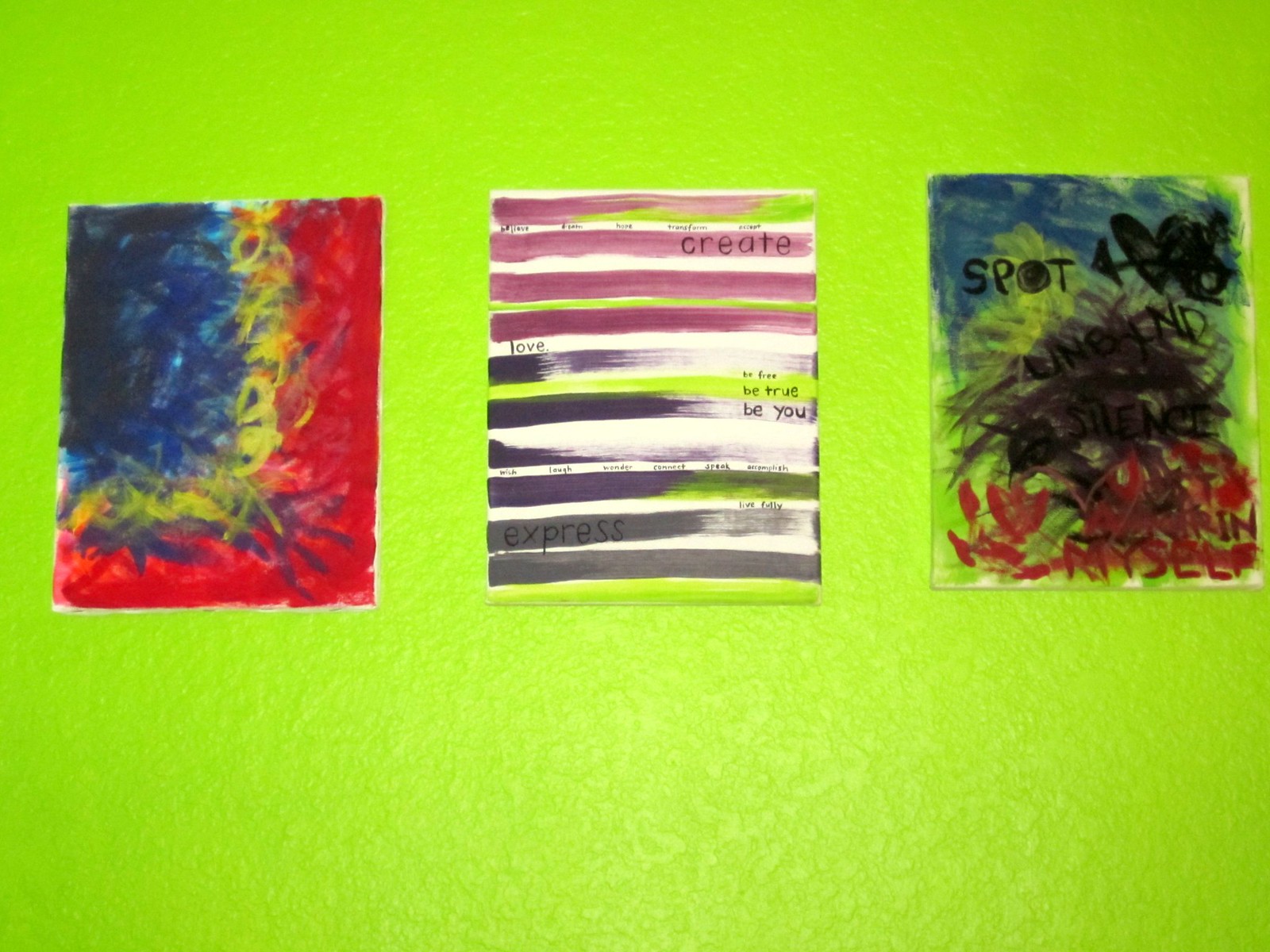The image showcases three unique abstract paintings displayed side-by-side against a vibrant lime green wall. The first painting on the left conveys a finger painting style, characterized by a deep blue swath bordered by bright yellow swirls that transition into orange. The rest of the painting features a chaotic mix of deep red, purple, and black tendrils extending towards the center, with a notable inverted 'L' shape in red positioned along the bottom right.

The middle painting is more structured, presenting a series of horizontal brushstrokes in varying colors. It begins with purple strokes at the top, which transition into darker shades of blue and almost black, with hints of green. This piece is adorned with several motivational words and phrases such as "create," "love," "be free," "be true," and "be you" inscribed across different stripes, imparting a message of inspiration and self-expression.

The third painting on the right exhibits a dynamic amalgamation of colors with finger-painted splotches of blue, yellow, green, black, and red. Amidst the abstract forms, a black heart pierced by an arrow stands out. Words like "spot," "unbind," "silence," and "myself" are scattered throughout the artwork, adding a layer of introspection to its vibrant chaos. All three paintings are neatly aligned in the upper-central portion of the lime green wall, creating a visually stimulating and thought-provoking display.